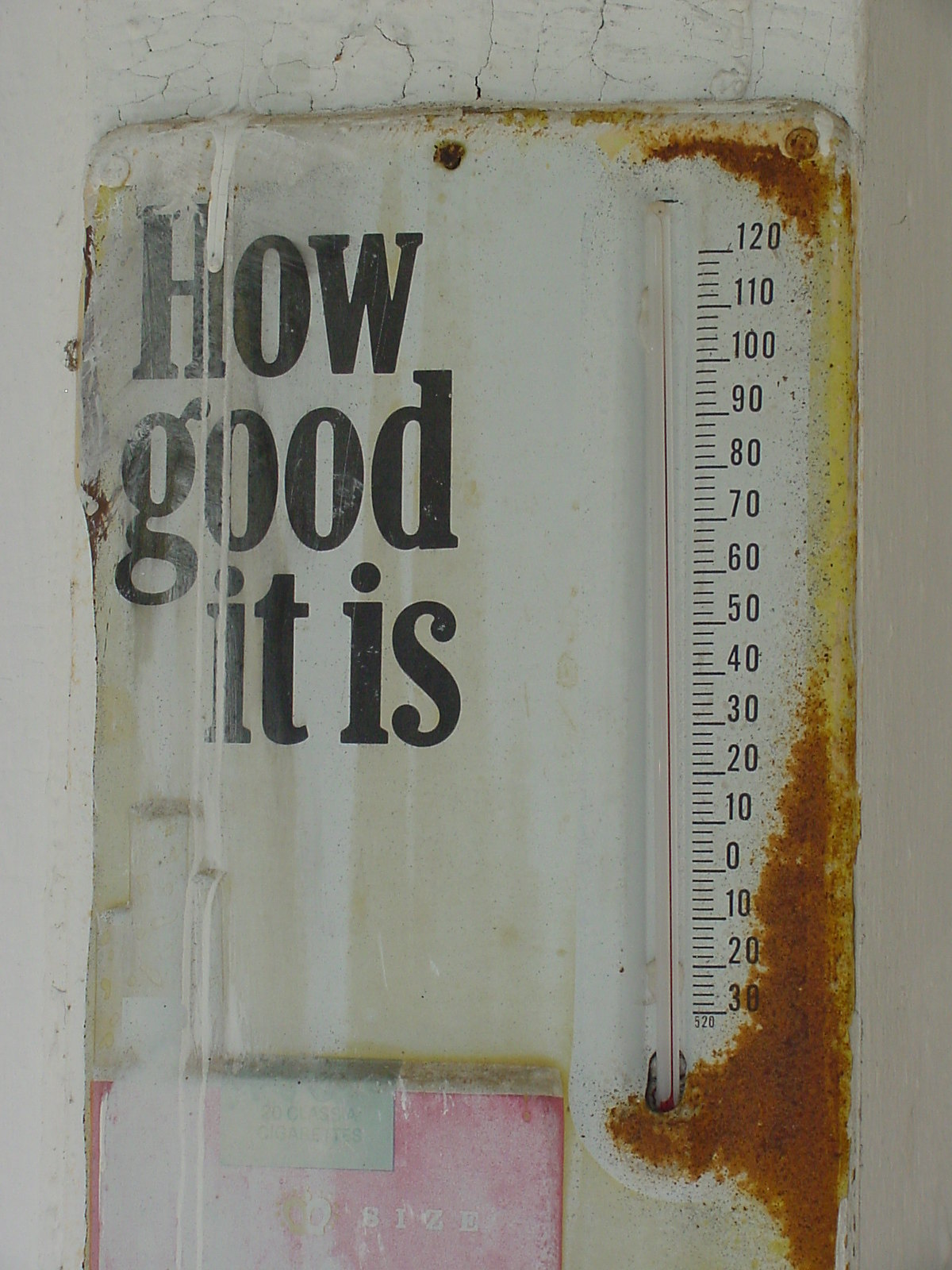A detailed examination of the image reveals a weathered metal sheet affixed to a wall, serving as some sort of poster. The sheet is secured with screws and is situated on a wall that shows visible signs of age, with pronounced cracks decorating its textured, white surface. The metal poster, which is mounted on the left side, is slightly bent about an inch inward at its edge, giving it a distressed appearance. Originally intended to be a cream color, the metal now looks uneven and faded. In the bottom section of the poster, there is a rectangular pink box, adding a touch of contrasting color to the otherwise muted palette.

On the right side of the poster, a prominently featured thermometer displays a temperature range from 30 to 120 degrees. The upper right corner of the thermometer is significantly corroded, exhibiting rust in various shades of brown, yellow, and orange. A yellow line runs vertically through this corroded section, accentuating the decay. Further rust streaks extend downward, growing thinner as they reach the bottom of the thermometer, yet still distinctly visible.